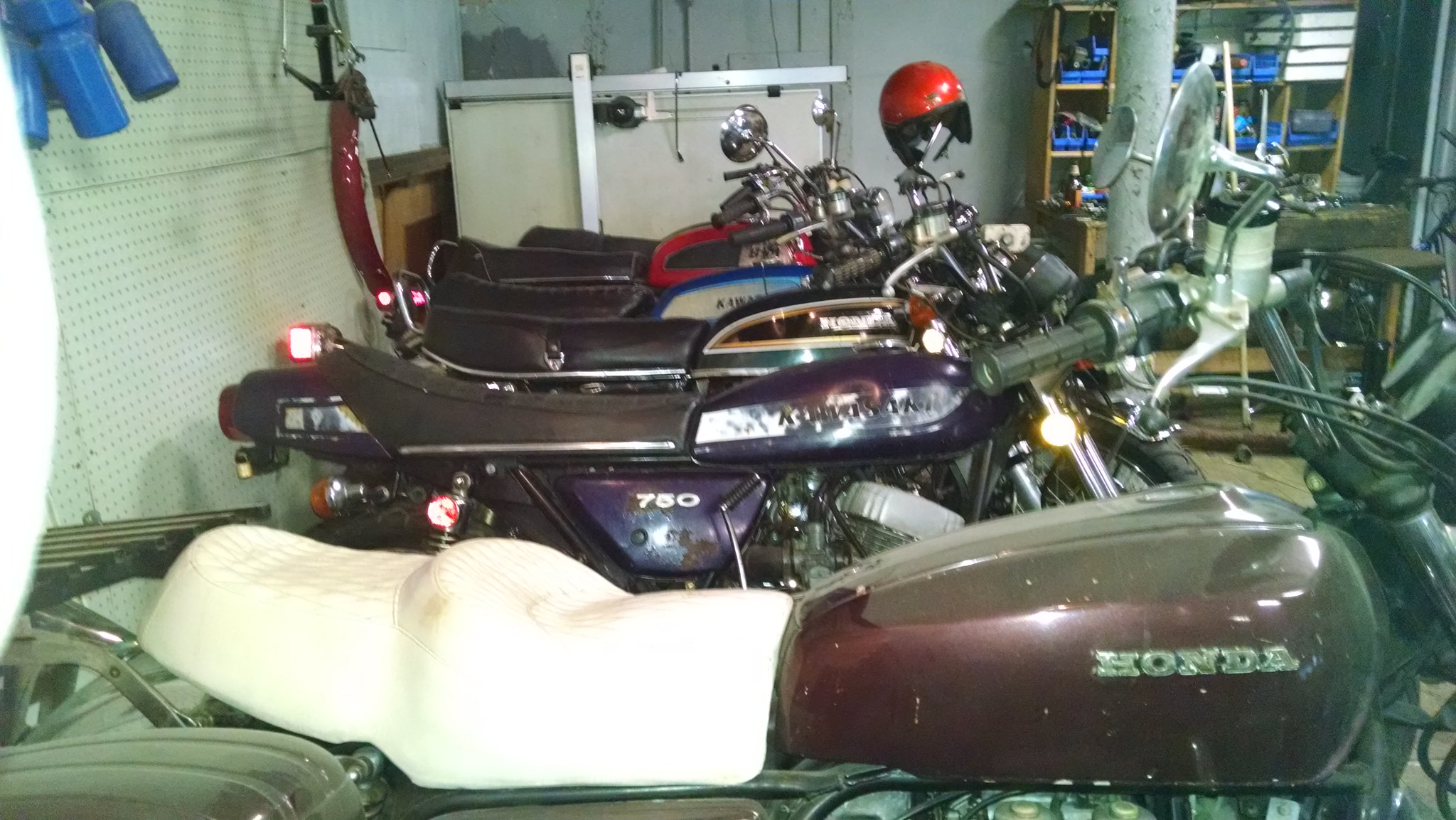The image is an amateur photograph capturing a lineup of classic motorbikes inside a gray-walled garage adorned with tools and a white desk against the left wall. A row of six motorbikes stretches from left to right, with the motorcycles facing sideways towards the right wall. Closest to the frame is a slightly blurry Honda showcasing a reddish-burgundy carrier shell and a white seat, with reflected lights on the tank. Following it is a Kawasaki 750, distinguishable by its blurred yet legible lettering, a running light, and a purple tank. Behind it, another Honda features a black case. The subsequent motorcycle is a Kawasaki with a bluish tank. Further back stands a motorbike with a black seat and a hard-to-read striped tank, and lastly, a red-cased motorbike adorned with a red helmet hanging on its handlebars. In the rear, a shelving unit with blue containers filled with parts completes the scene.